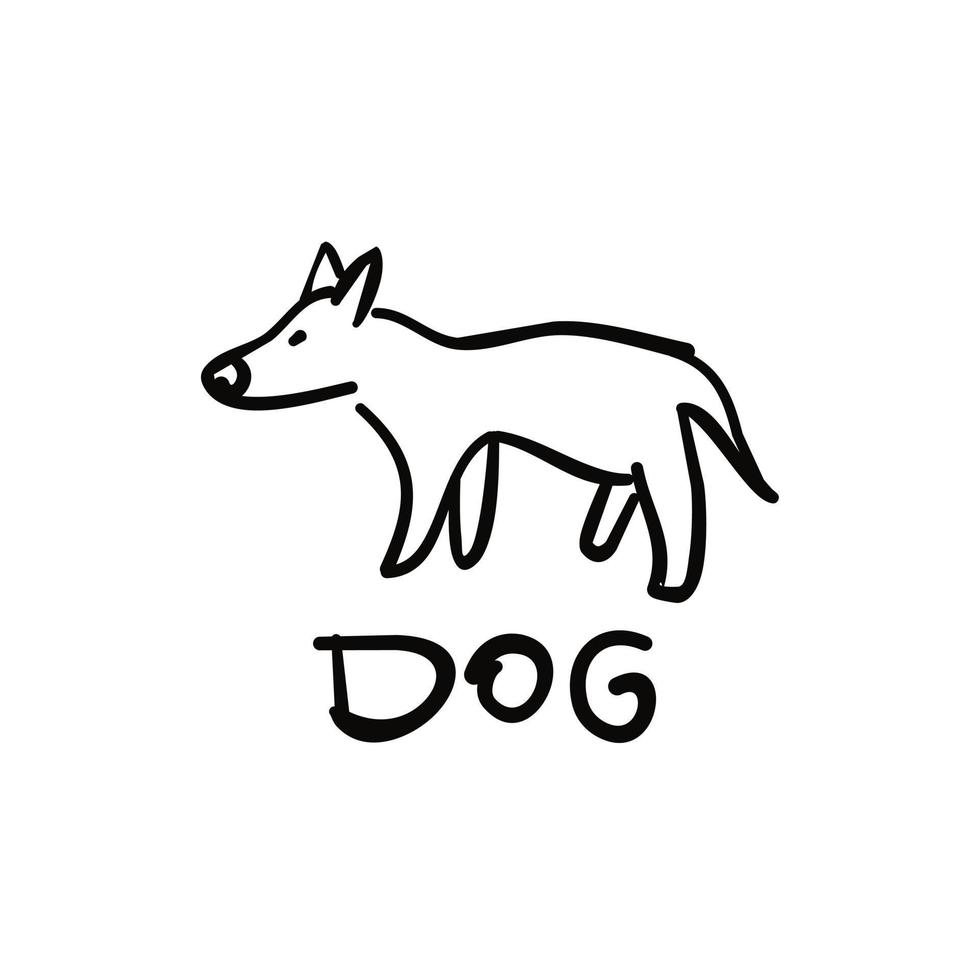The image is a freehand drawing depicted on a completely white background without any borders. The entire illustration is rendered using black lines, giving it a minimalist graphic style. 

The drawing showcases a dog standing on all four legs, facing towards the left. The dog features pointy ears, a long snout with a big nose, and a single dot for an eye, giving it a simplistic but expressive look. Its tail is pointed, drawn with a single line that extends towards the bottom right corner of the image. The front left leg is positioned forward while the back left leg is behind, creating a walking stance. 

Below the dog, there is a handwritten text in large, all-capital letters that reads "DOG," also in dark black color, matching the style of the drawing. The overall dimensions of the drawing are estimated to be around two inches high and three inches wide, giving it a compact, yet detailed appearance.